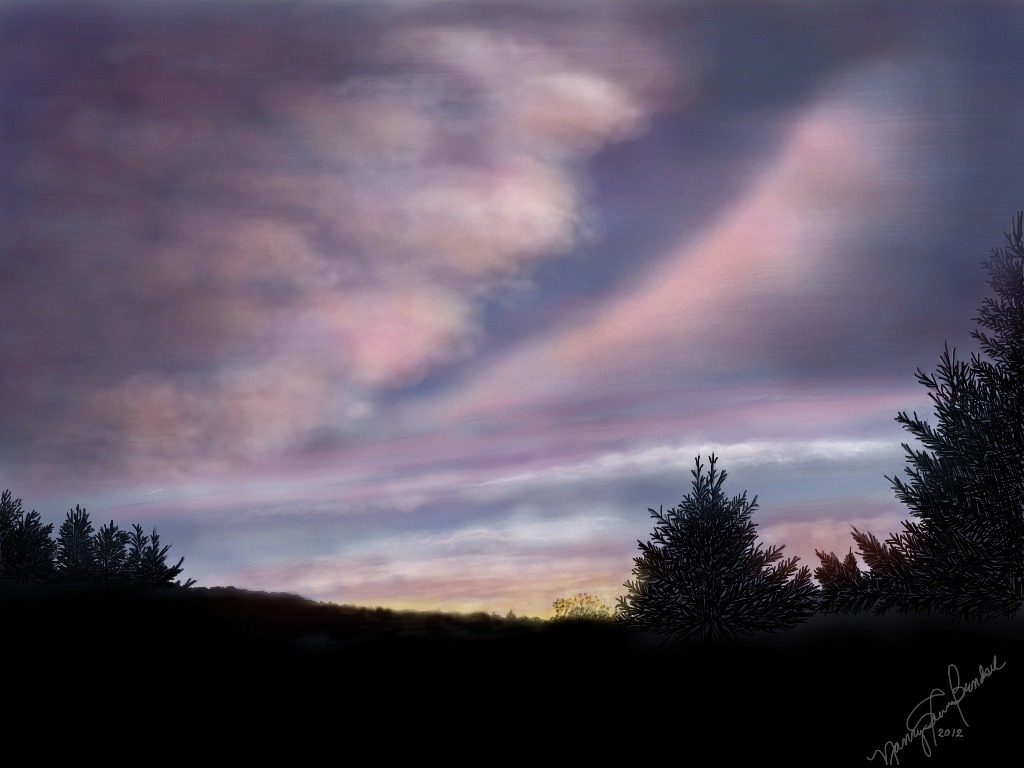This painting captures an evocative landscape during sunset. The upper three-quarters to four-fifths of the image is dominated by a dramatic sky filled with textured clouds. The background of the sky at the top showcases a deep dusty blue, gradually transitioning to a lighter blue as it descends towards the middle. Near the horizon, soft yellow hues hint at the retreating sun. The clouds themselves are a vibrant mix of whites, grays, pinks, purples, and oranges, creating a rich tapestry of colors and forms. They drift in various directions, giving rise to an array of shapes and patterns. In the bottom quarter of the image, a silhouetted strip of land is visible, adorned with a scattering of bushy and pine-like trees, adding depth and a sense of stillness to the scene below the dynamic sky.